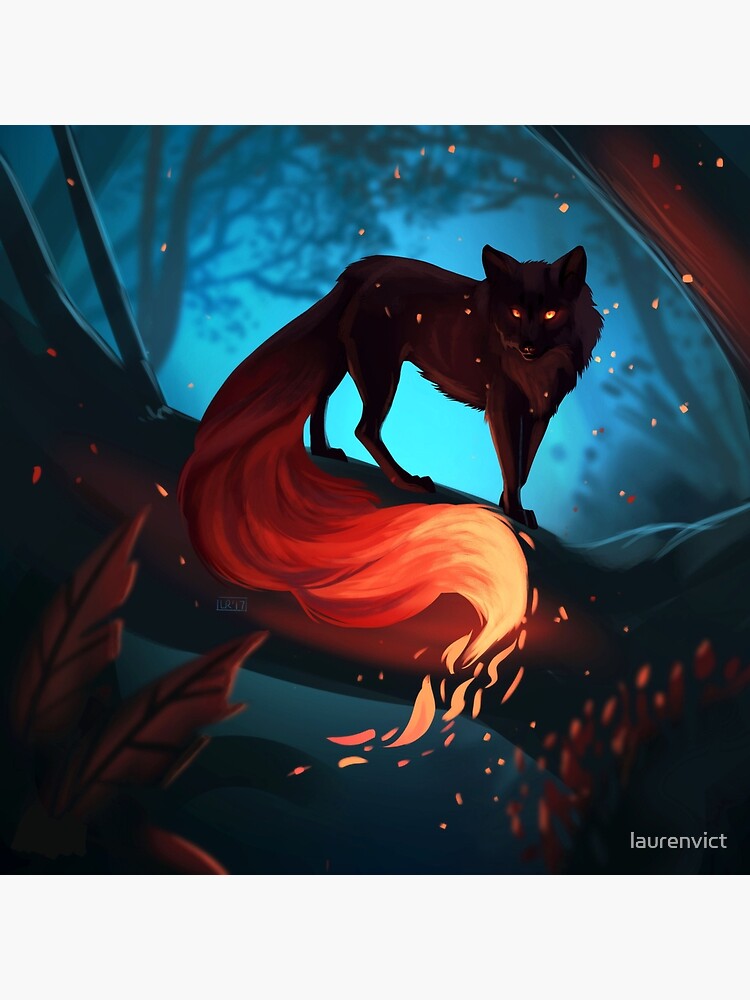This digital art piece depicts an enigmatic creature, possibly a wolf or fox, perched prominently on a horizontally positioned, wide tree branch that extends from the lower right to the upper left of the image. The creature's dark form is illuminated by its mesmerizing, glowing orange eyes, which gaze directly at the viewer. Its tail is notably oversized and transitions into vivid, flame-like appendages at the end, emitting a fiery glow that casts a warm light on its surroundings.

The background is a dynamic interplay of contrasting blue hues, punctuated by shadowy silhouettes of forest elements such as tree trunks and branches. This gives a sense of depth and immersion into a mystical, twilight forest scene. The lower left corner of the image is dotted with large leaves, their tips tinged with orange from the illumination caused by the creature's fiery tail. Additionally, the air around the creature contains small, glowing orange embers or sparks, adding to the mystical atmosphere.

The piece also features the text "Lorin vikt" in small white print in the lower right corner, adding a hint of subtlety to the overall composition. This artwork's intricate details and ethereal lighting evoke a sense of mystery and fantasy, reminiscent of scenes from a video game.